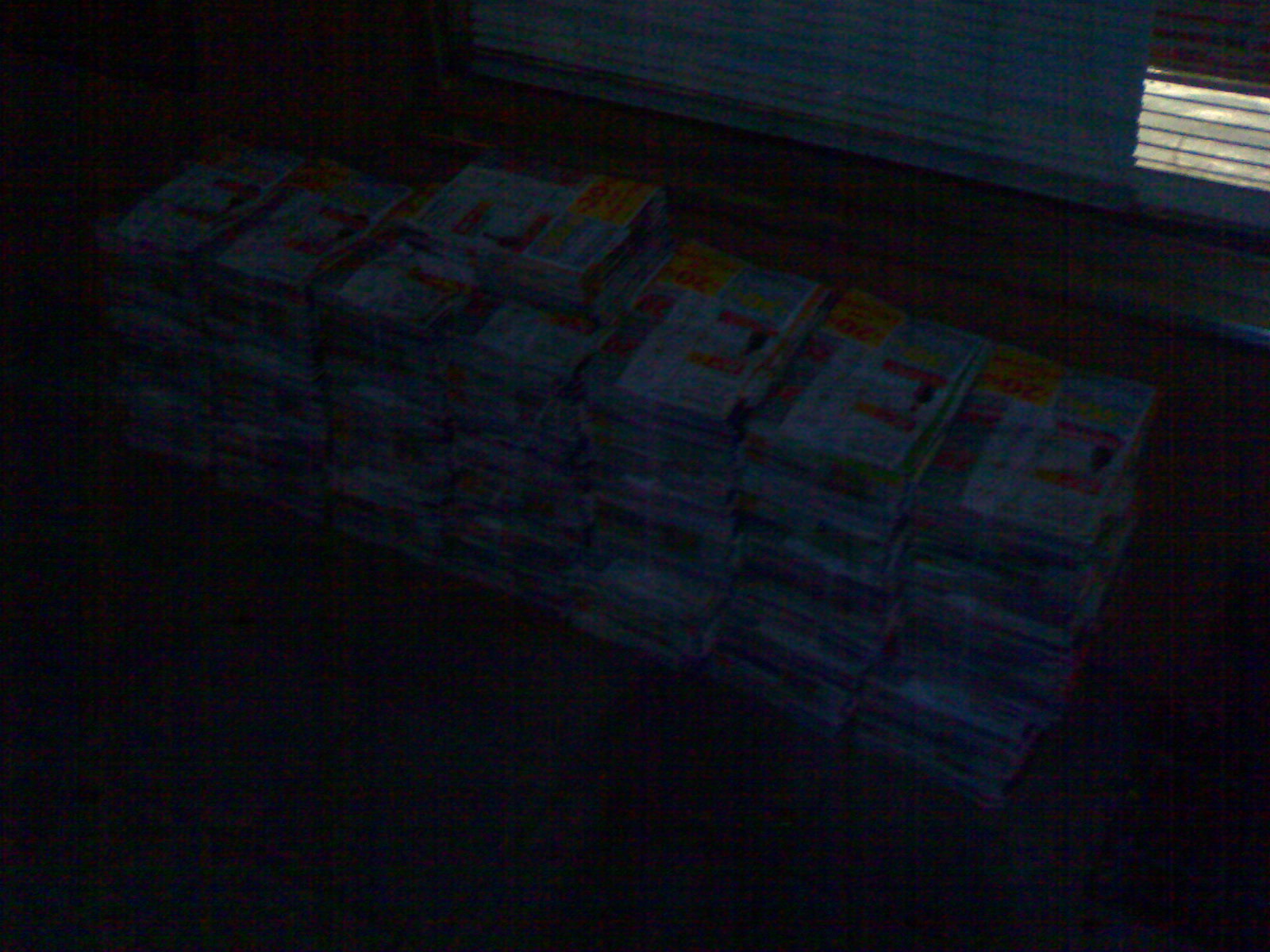The image is an extremely dark photograph depicting about seven stacks of newspapers, or possibly catalogs, bound in plastic, indicating bulk delivery. These stacks are positioned side by side, starting from the upper left corner and descending towards the bottom right of the frame. In the center, one bundle is notably placed sideways atop the stacks. The scene likely captures a pre-dawn delivery, as the bundles are set outside, possibly on a road or sidewalk, against the backdrop of a window or a gated store. In the top right corner, blinds can be seen, adding to the overall dim ambiance of the image.